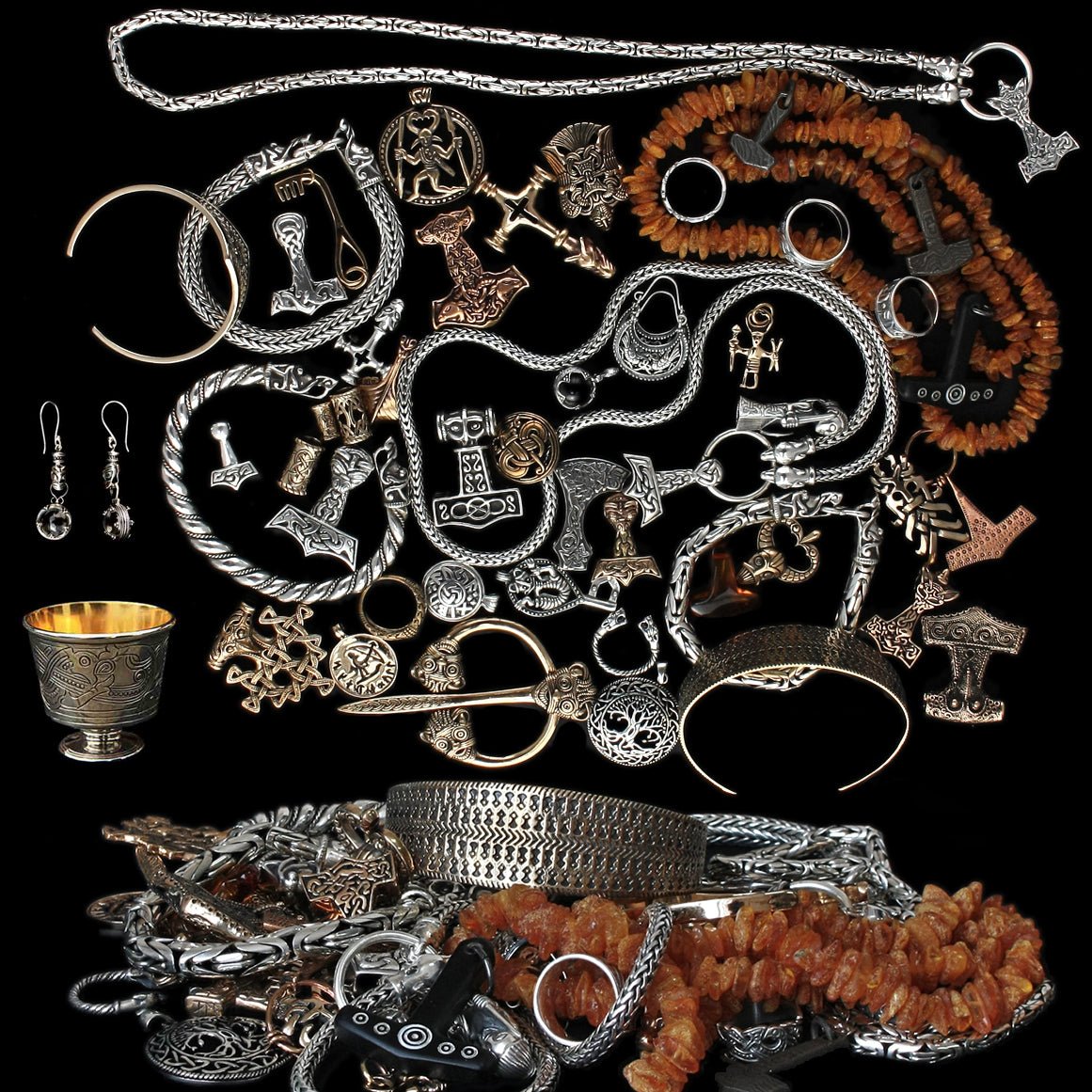The square image features a dark black background and is densely covered with an array of silver and gold jewelry, evoking a sense of medieval-era adornments or pirate treasure. At the top, a long silver chain with a pendant lies horizontally, while below it, a variety of silver bracelets and bangles, some braided and some with clasps, are arranged nearly on top of each other. In the middle, several more silver chains and bracelets intermingle, punctuated by hook earrings on the far left. Brown beads, possibly forming part of a necklace, are interspersed with silver rings and other baubles, one of which cascades across the collection. Towards the bottom, the jewelry becomes a tangled mass, making individual pieces indistinguishable. A tin with a golden item inside also appears among the scattered pendants, rings, and other trinkets, adding to the eclectic assortment of what could be considered lost treasure or historical artifacts.